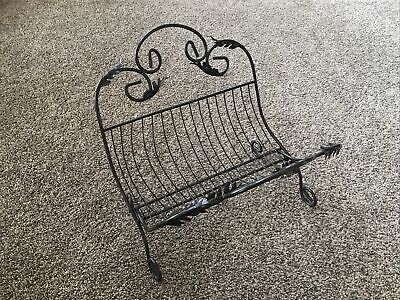This is a photograph of a black wrought iron wood holder, designed to cradle firewood, reminiscent of a baby cradle. It features curved handles at the top with decorative wrought iron leaves, and is supported by sturdy, curved legs with curly-Q loops at the bottom. The body of the holder consists of curved support wire ribbing, providing ample space to stack wood securely. The item is detailed with swirling patterns and sits on a tan carpet, enhancing its decorative appeal. A fireplace poker is also part of this scene, sticking out from the bottom, confirming its use near a fireplace. The setup combines functionality with intricate design, making it as aesthetically pleasing as it is practical for holding firewood.